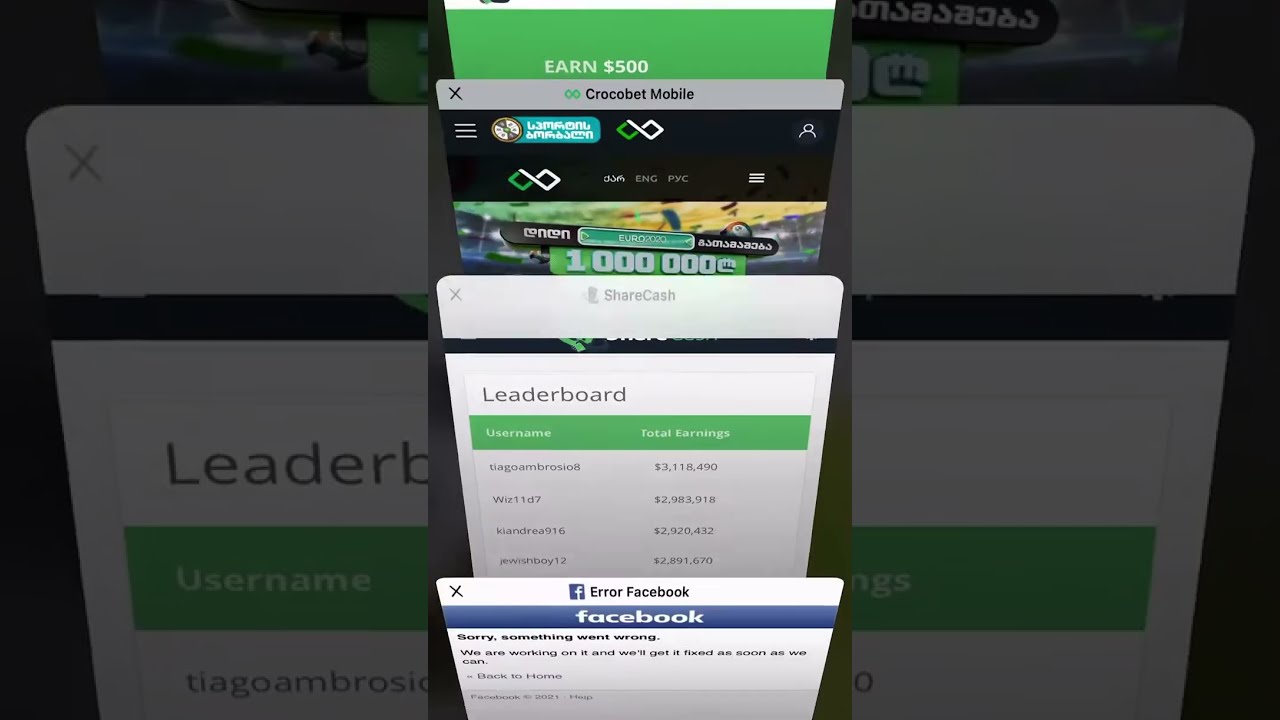The image is a wide rectangular composition, featuring a primary screenshot of a phone screen in the center. On either side, there are two darker, zoomed-in sections of the same screenshot, each focusing on different edges of the central image. The main screenshot displays a light gray background with several spaced-apart white rectangles stacked vertically. At the top, part of a black bar with white and green font is visible. Directly below, a white rectangle reads, "Use this link to share on Facebook," accompanied by a small Facebook icon. Beneath this, a clickable green rectangle with white text states, "$30 Surveys and Apps." Further down, there are four white rectangles, each featuring a colored circle on the left and text on the right. The first rectangle shows a blue circle with a white arrow, next to "Clicks 33" in black font. The second rectangle contains a red circle with an icon resembling people or a present, with "Referrals 2" to its right. The third rectangle features a green circle with the numbers 1, 2, and 3 inside, and "Tasks 7" written beside it. The last rectangle displays an orange circle with a white dollar sign, with "Earnings $321" to the right. Toward the bottom, partially cut-off text begins with "Warning when confirming payments if our..."